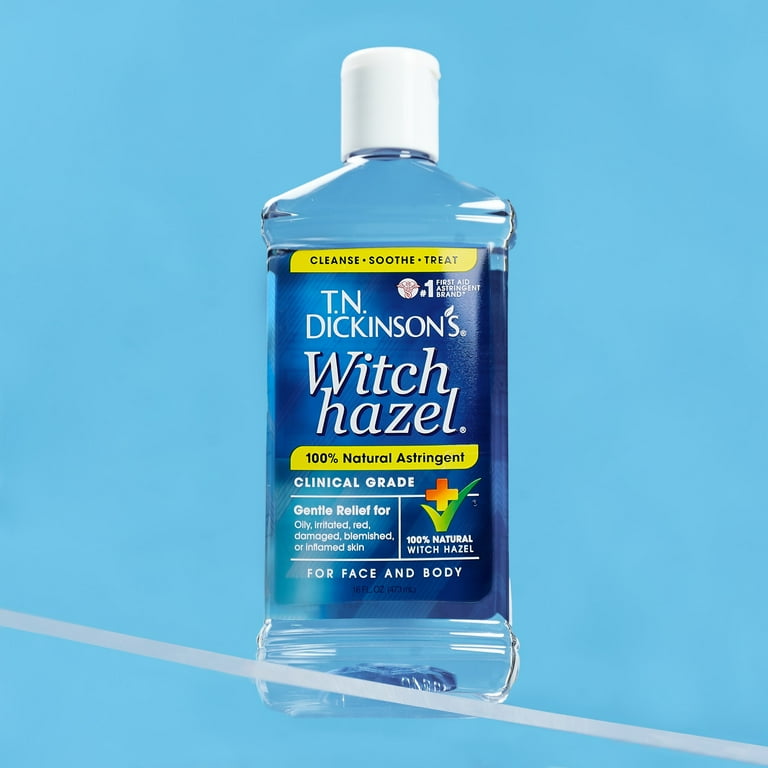This image features a 16-fluid-ounce bottle of T.N. Dickinson's Witch Hazel, a clinical-grade cleansing product designed for both the face and body. The bottle, made of clear plastic with a white twist cap, contains clear liquid. Its label is predominantly navy blue with sections accented in yellow text bars. At the top, the label reads "Cleanse, Soothe, Treat" in black text within a yellow border. Directly below, it states the brand name "T.N. Dickinson's Witch Hazel" in white text. Further down, a yellow oval with black text highlights that the product is a "100% Natural Astringent." Under this, additional information notes the product's clinical grade, detailing its gentle relief properties for issues such as oily, irritated, red, damaged, blemished, or inflamed skin. The background of the image is a light sky blue with a diagonal white stripe across the bottom that slightly overlaps the bottle, adding a modern, dynamic touch to the presentation.